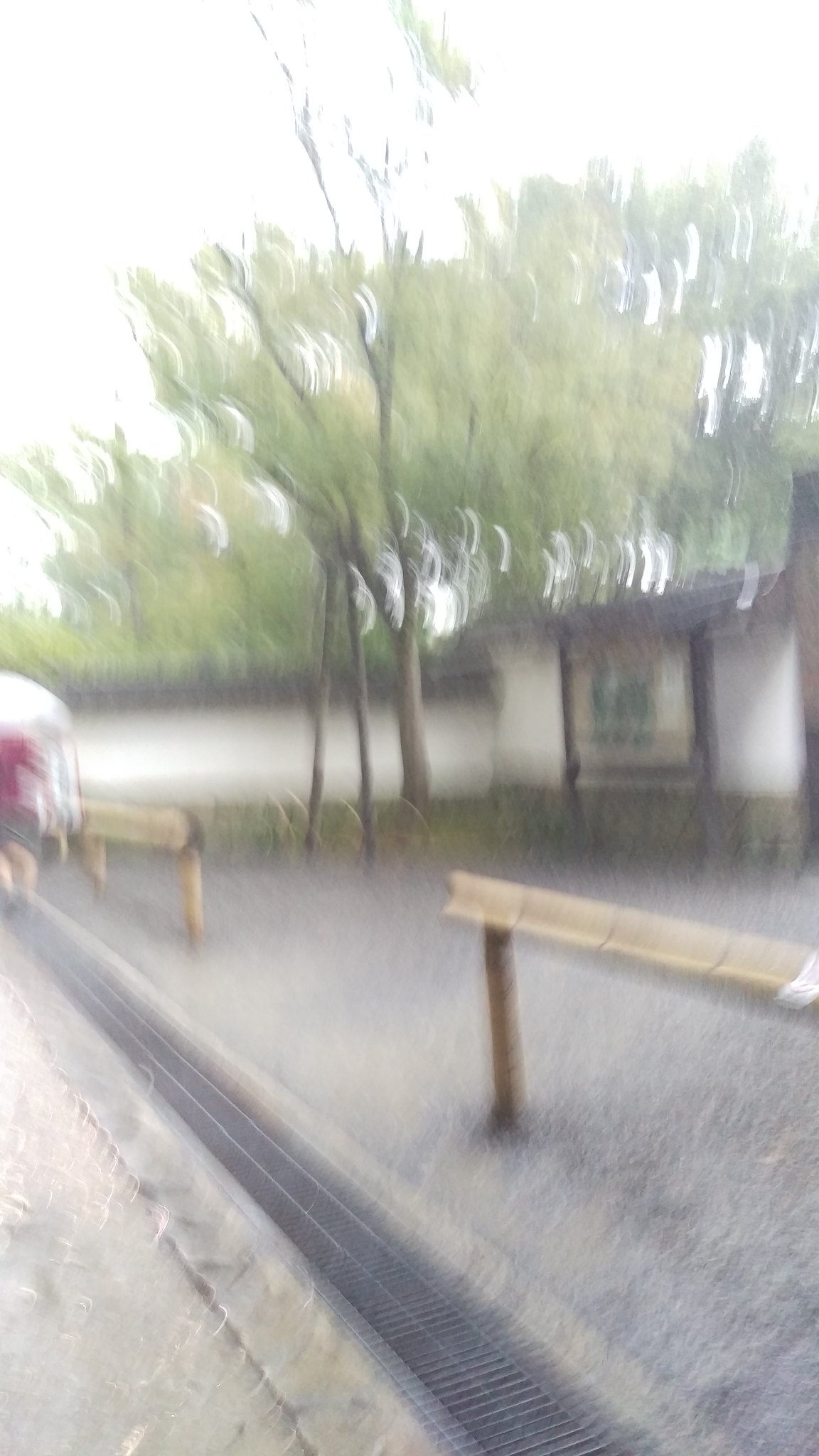The image resembles a painting, capturing a streetscape scene. In the foreground, a curb runs alongside the road with a pavement featuring interrupted railings. On the far left, a figure or object dressed in a red top and grey bottoms can be seen. Beyond the pavement lies a long, low, white building accompanied by a patch of green grass, offering a serene backdrop. Delicate, spindly trees stand in front of the building and continue behind it, adding depth and a sense of continuity to the scene. Further in the background, a long, white wall stretches across, with additional trees rising behind it, completing the layered, picturesque landscape.